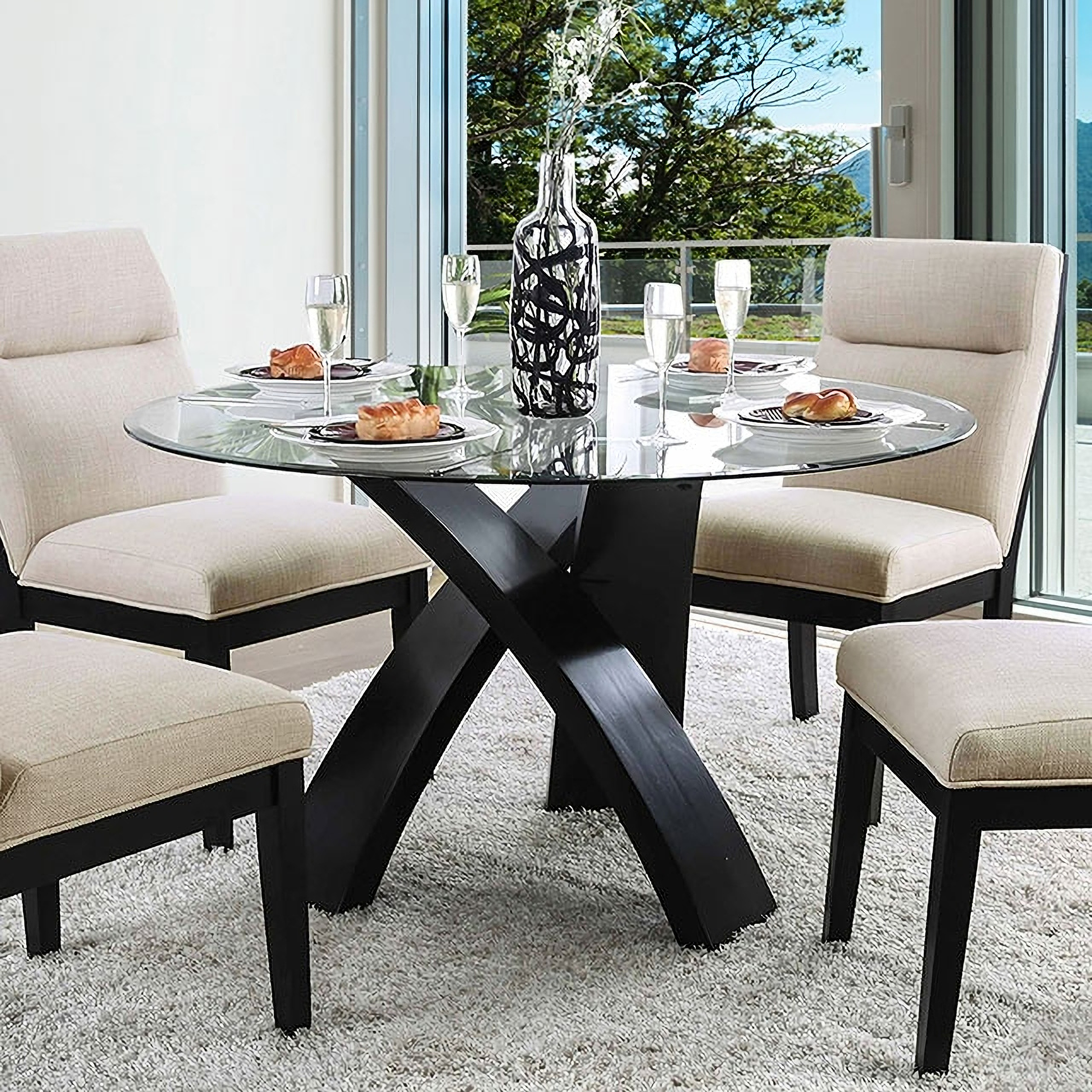This indoor image showcases a well-appointed dining area featuring a circular glass-top table supported by three sculptural, black-painted wooden posts arranged in a twisting triangle pattern. The table is elegantly set with four white plates containing brown pastries, accompanied by silverware and bubbling champagne glasses. At the center of the table stands a clear glass vase with intricate black lines, holding white flowers. Surrounding the table are beige-cushioned chairs with black trim and legs. The dining area is situated on a soft gray shag carpet, while the soft white beige walls create a warm ambiance. In the background, a sliding patio door with a Levolor curtain offers a picturesque view. Beyond the glass, a well-manicured lawn is bordered by a gray or white fence, with lush trees and a majestic mountain range against a blue sky speckled with white clouds.